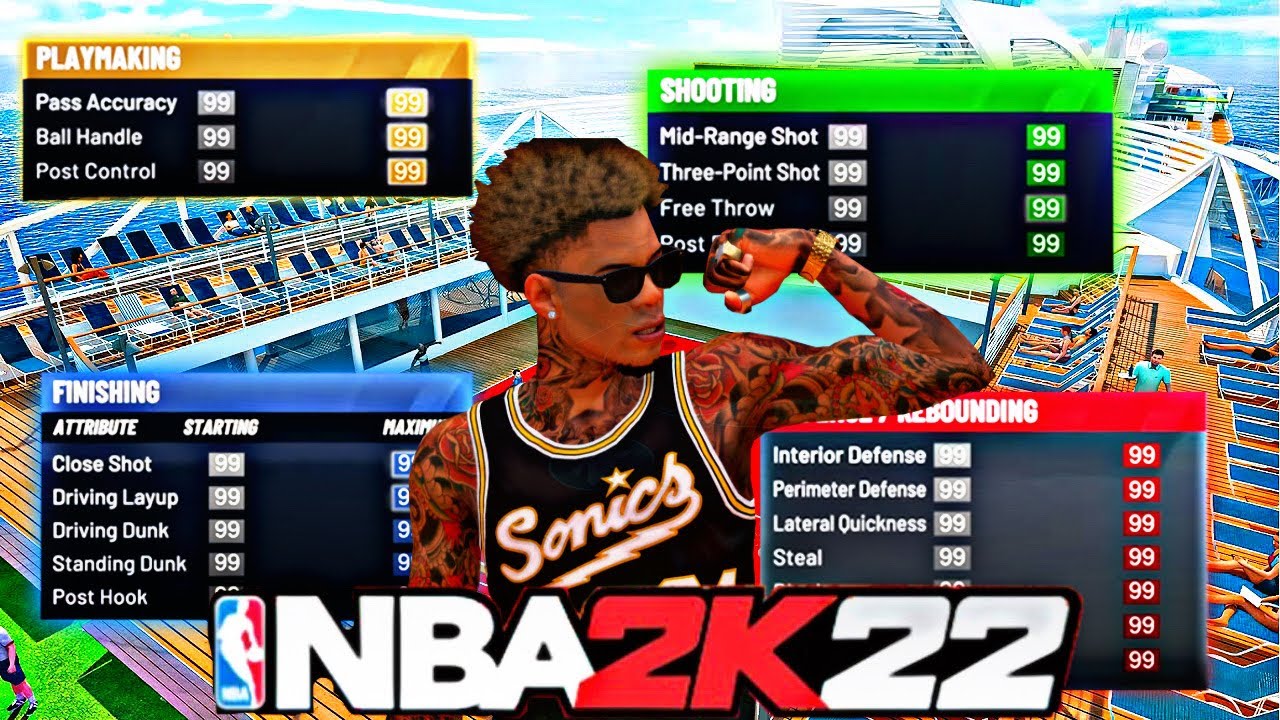The image features a screenshot from the video game NBA 2K22, characterized by its wide aspect ratio, roughly twice as wide as it is tall. Dominating the bottom portion of the image is the distinctive NBA 2K22 logo. The iconic NBA logo, a white silhouette of a basketball player on a blue and red background, is situated to the left side and is accompanied by the text "NBA 2K22," with "NBA" in white, "2K" in red, and "22" in white.

Central to the image is an in-game character, an African American man depicted from his chest upward. He is heavily tattooed from his neck down to the ends of his arms, showcasing intricate body art. The character sports afro-like hair and wears black sunglasses, and is posed flexing his left arm to show his bicep.

In the upper left corner, there is a chart section with a yellow-gold banner headlined "Playmaking." Surrounding it are additional charts labeled "Shooting," "Finishing," and an unreadable fourth category, all of which help to contextualize the player's skills within the game.